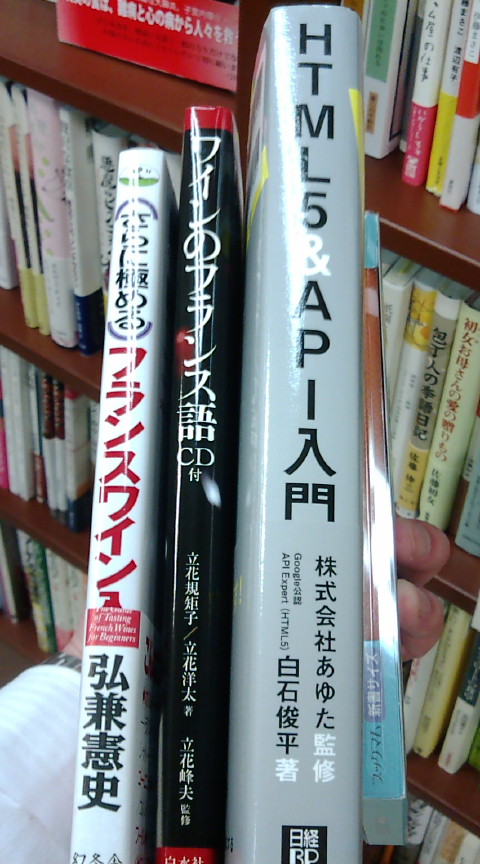This image captures a close-up of a hand holding four books against a backdrop of densely packed bookshelves in what appears to be a library or bookstore. The bookshelves are filled with various books, giving the setting a bustling, scholarly ambiance. The books, held to display their spines to the camera, all feature predominantly Asian characters, presumably Japanese. Starting from the left, the first book has a white spine with red and black characters and contains partially visible English text saying "Tasting French Wines for Beginners." Next to it is a black book with white Japanese characters and a small red accent, also including the English letters "CD." The third book, and by far the thickest, is a gray spine textbook that prominently reads "HTML5" and "API" in English, along with additional text "Google API Expert HTML5," supplemented by Japanese characters. The fourth and final book, partially obscured by the third, has a narrow spine with an orange and light blue design, but the glare on its cover makes it difficult to identify any characters. All books have a reflective surface, adding a layer of sheen that enhances the vibrant and diverse array of spines captured in the image.